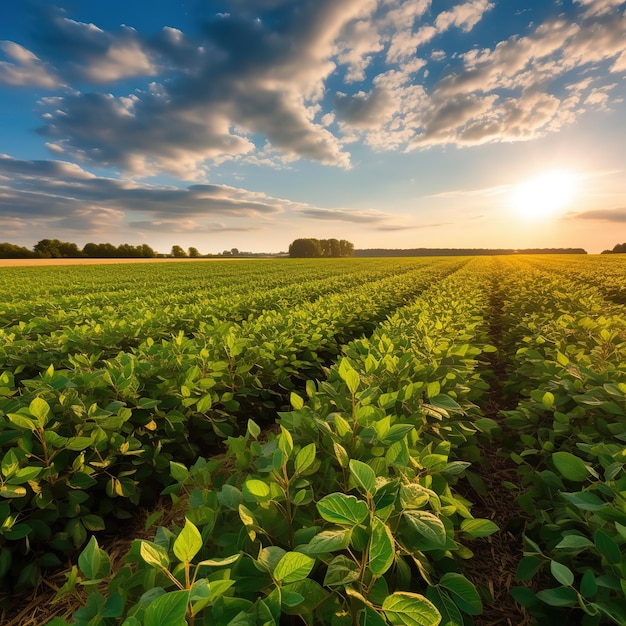A photograph of a farmer's crop field captures an expansive scene of verdant rows in the early stages of growth. The neatly aligned crops run diagonally from the lower left corner to the upper right, creating a repetitive pattern of lush green and varying shades. A dirt trail weaves alongside the center row, adding an earthy contrast. In the background, a cluster of trees, primarily brown with sparse green foliage, stands against a horizon framed by a more distant and thin tree line. The sky above showcases a picturesque mix of billowy, white, and slightly gray clouds with streaks of peach near the horizon, hinting at either sunrise or mid-afternoon light. The sun, positioned low in the sky, casts a warm, yellowish hue over the field, enhancing the early growth's vibrant green and creating a sense of serenity on this lovely summer day.